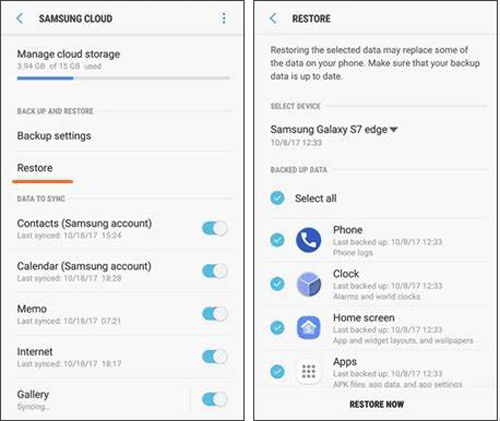The image depicts two screenshots from a Samsung Galaxy S7 Edge phone, showcasing the Samsung Cloud interface. The left screenshot titled "Samsung Cloud" shows the "Manage Cloud Storage" screen, indicating that approximately two-thirds of the storage is utilized. Below are options like "Backup and Restore" and "Add Backup Settings," accompanied by a "Restore" button, highlighted in orange. Additional details include a list of data to sync with slide buttons for toggling items like Contacts, Calendar, Memo, Internet, and Gallery, all of which are turned on.

The right screenshot displays the "Restore" screen, which warns: "Restoring the selected data may replace some of the data on your phone. Make sure that your backup data is up to date." The name of the device, Samsung Galaxy S7 Edge, is shown, with a date stamp of October 8, 2017, and the exact backup time mentioned. The backup data selection includes all categories like phone, clock, home screen, and apps, all checked off. A "Restore Now" button is available for initiating the process.